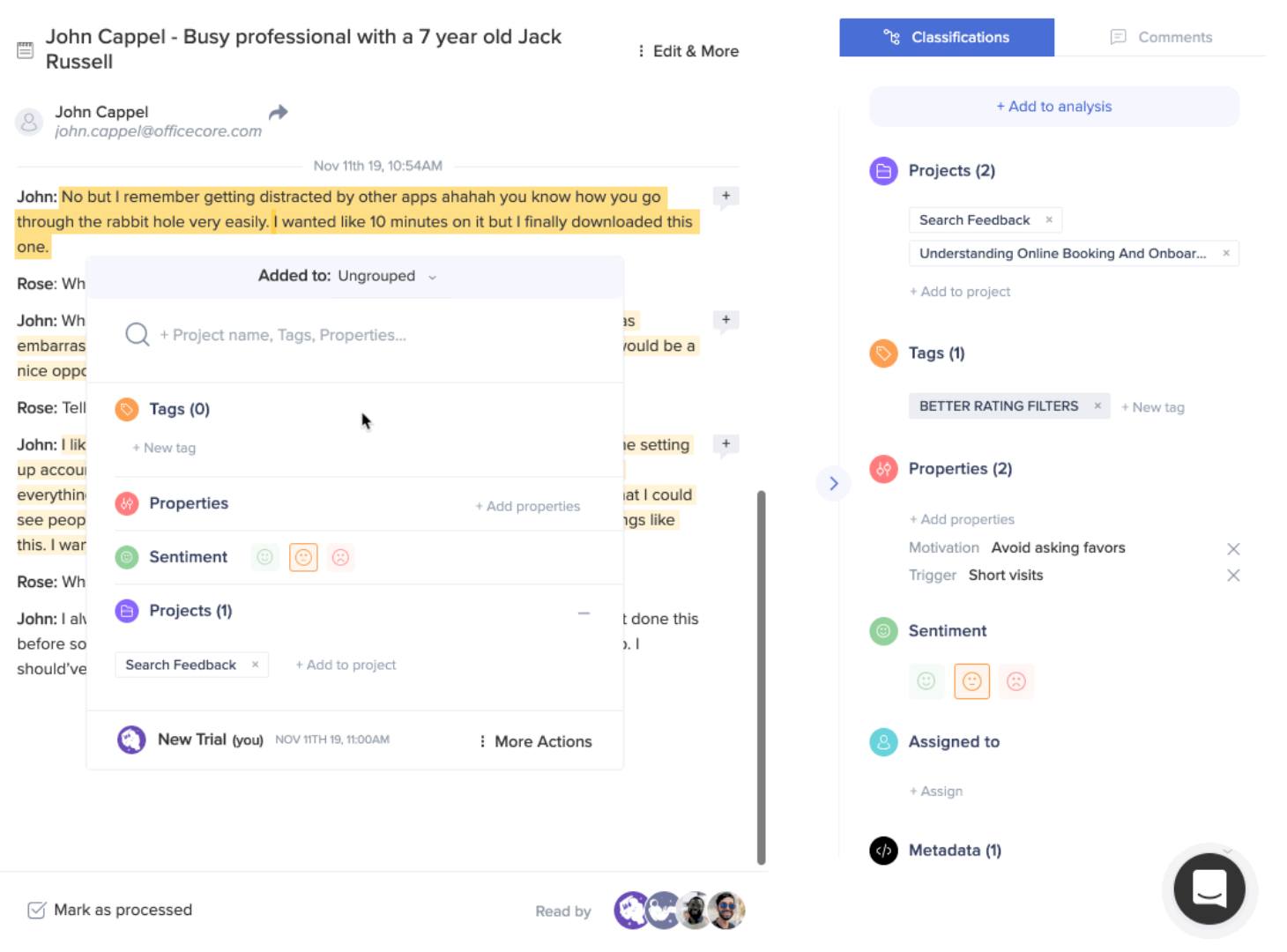**Detailed Caption:**

The image is a screenshot of a web page displaying a conversation thread. The webpage has a white background. At the top left, the header reads "John Capel - Busy Professional with a Seven-Year-Old Jack Russell," where "Jack Russell" refers to his dog. To the right of his name, there are options labeled "Edit" and "More."

Below the header, John Capel's contact information is listed as "John Capel, john.capel@officecore.com." Just beneath, there's a timestamp indicating "November 11, 2019, 10:54 a.m."

The message from John, highlighted in light orange, starts with "John: No, but I remember getting distracted by other apps hahaha. You know, you go through the rabbit hole very easily. I wanted like 10 minutes on it, but I finally downloaded this one."

Following this, there are excerpts of a conversation including:
- John: "WH [remaining text not visible] ... embarrassed ... opportunity"
- Rose: "Tell [remaining text not visible]"
- John: "[something about accounting and everything]"

A notification overlay partially obscures the conversation, stating "Added to ungrouped" with various icons labeled "Tags," "Icon for properties," "Icon sentiment," and "Icon projects" with a "(1)" in parentheses. Additional icons include "Search," "Feedback," and "New trial," followed by "More actions."

At the bottom of the screen, there are further details:
- "Mark as processed"
- "Read by" with four icons, including animated objects with a white and purple background, and two people: one appears to be a black man with a beard, and the other a white man with a beard and sunglasses.

On the right side of the screen, there are headers and options like:
- "Classifications"
- "Comments"
- "Add to analysis"
- "Projects" with a count of 2
- "Search feedback"
- "Understanding"
- "Online booking"
- "Onboarding" (likely text cut-off)
- "Tags"
- "Properties"
- "Sentiment"
- "Assigned to"
- "Metadata"